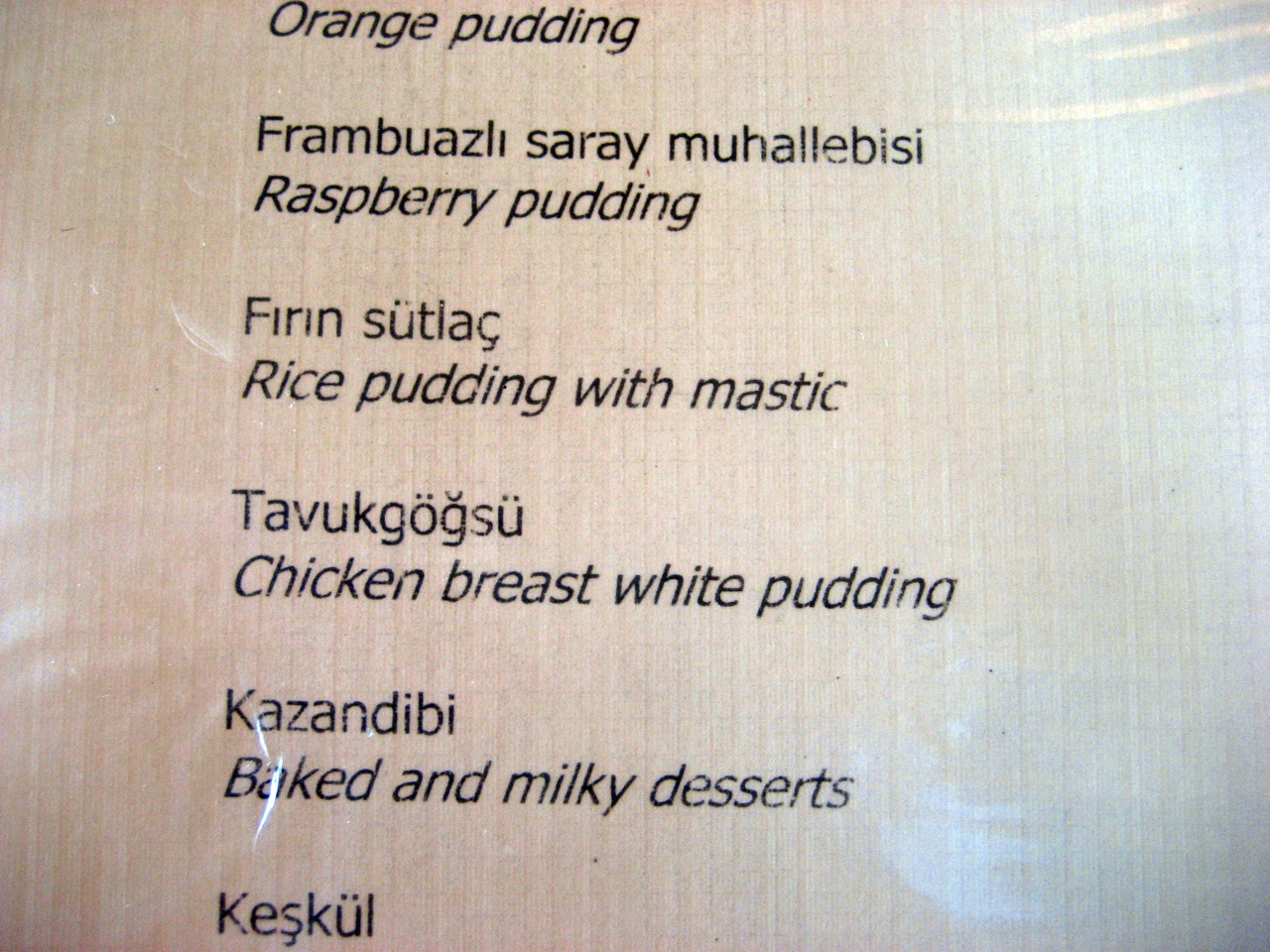The photograph depicts a close-up view of a section of a menu, likely from a restaurant. The menu is printed on textured white paper and features a list of dishes written in black ink. The legible items on the menu include "Orange Pudding," "Raspberry Pudding," "Rice Pudding with Mastic," "Chicken Breast," "White Pudding," and various types of baked and milky desserts. Additionally, there is text in a second, unidentified language. Due to the tight crop of the image, the surrounding setting is not visible, leaving the exact context within a restaurant or at an event unclear.